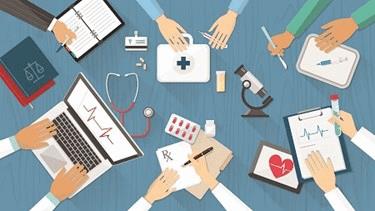This colorful, cartoon-style illustration on a dark blue background showcases six sets of hands engaging with various medical tools and items. The hands are depicted in different positions and attire, reflecting a variety of roles within a medical setting. In the upper left, a hand writes in a planner, while in the top center, another hand hovers over a first aid kit with a thermometer in the left hand. To the top right, a left hand touches a tray with a syringe, and the right hand holds a scalpel. The hands in the bottom right are focused on a medical chart, with one holding a test tube. Directly below that, another hand writes on a prescription pad, accompanied by a packet of pills and a manila folder. The bottom left features hands typing on a laptop displaying an EKG. Scattered across the table are additional medical items, including a stethoscope, an ID badge, several pill bottles, and a microscope. The individuals are dressed in various outfits, such as white long-sleeved shirts, a suit jacket, and colorful lab coats, emphasizing the collaborative environment of the scene.